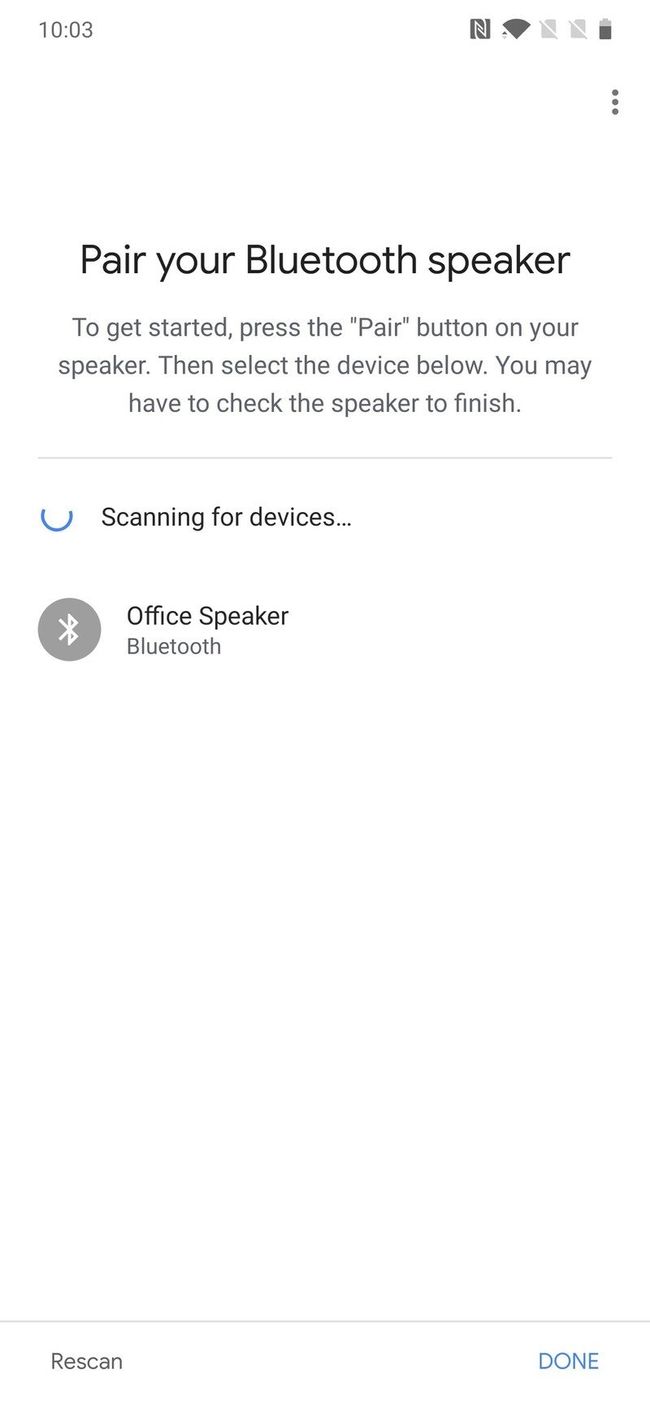The screenshot depicts a mobile phone interface detailing the process for pairing a Bluetooth speaker. The page is currently in scan mode, indicated by the message "scanning for devices." At the top, the header reads "Pair Your Bluetooth Speaker," followed by instructions: "To get started, press the pair button on your speaker, and select the device below. You may have to check the speaker to finish."

The interface shows an ongoing scan, with a Bluetooth icon and a scanning indicator prominently displayed. It has successfully identified "Office Speaker Bluetooth," which appears as an available device. At the bottom of the screen, there are two buttons labeled "Rescan" and "Done." The rest of the screen is minimalistic, with empty spaces typical of app pages awaiting user interaction. The layout reflects a simple and user-friendly design, optimized to guide users through the pairing process efficiently.